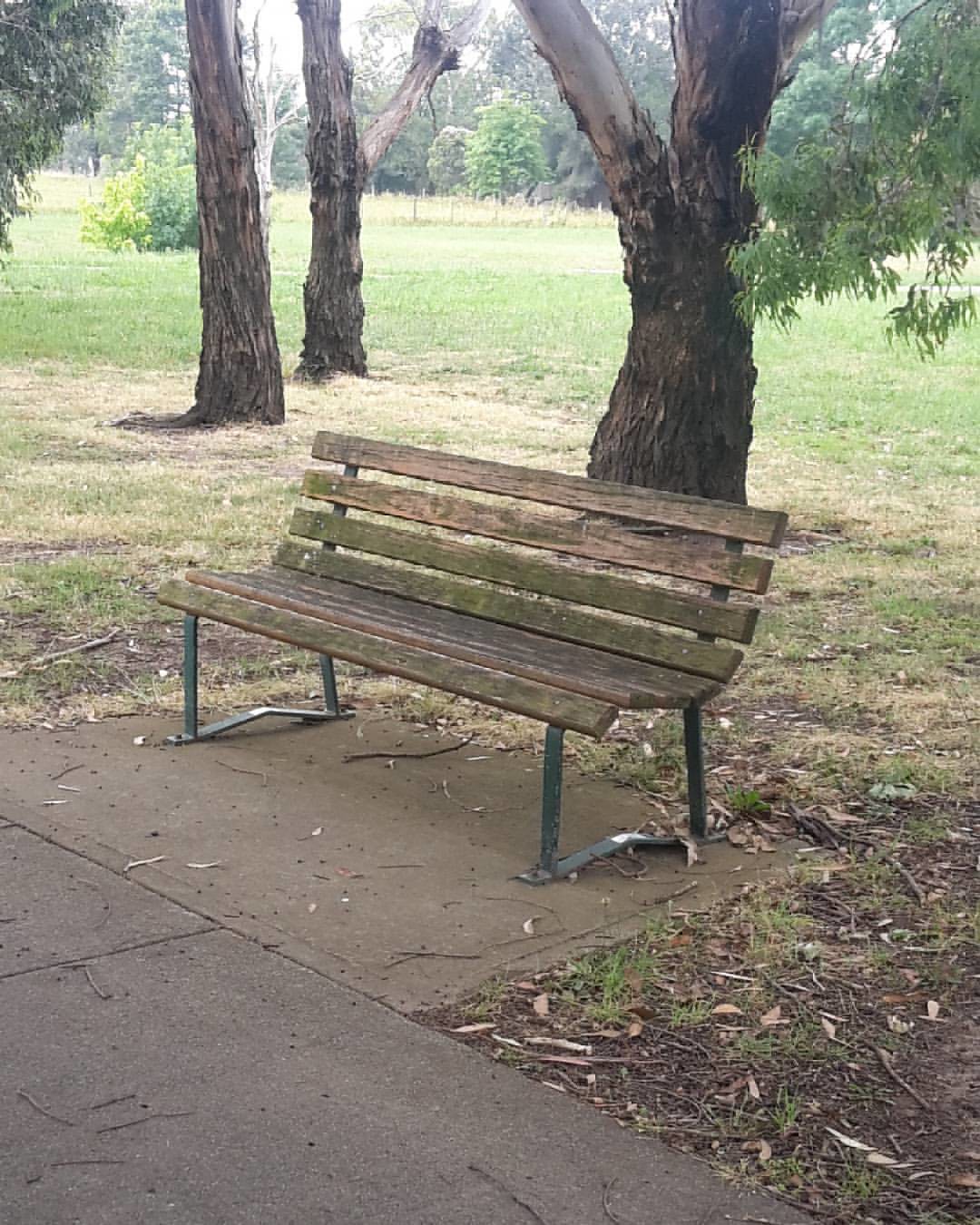In this daytime image, a weathered park bench is prominently featured, resting on a light brown concrete patch in a spacious park. The bench is composed of vertical wooden slats with a greenish tint, likely due to moss, indicating its age and lack of maintenance. It is supported by two sturdy gray metal legs connected by a horizontal metal bar for added stability. The bench is positioned adjacent to a gray concrete walkway. Surrounding the bench, the ground is covered with a mix of darker green grass and faded white areas with wood chips, scattered with small branches. In the background, several large trees with dark brown trunks and a mixture of bare branches and green leaves create a natural, scenic backdrop. One tree has a notable branch protruding upwards and displays hanging leaves. The overall scene suggests a peaceful, albeit slightly neglected park environment.